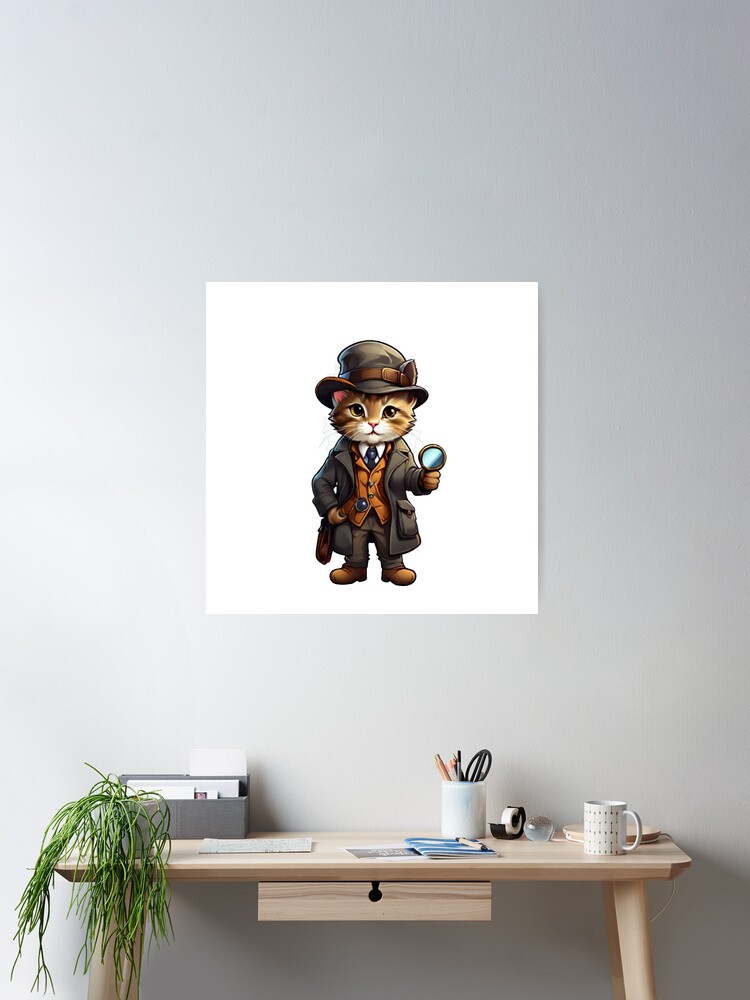The photograph depicts a modern, minimalist office setup featuring a light-coloured, natural wood desk, likely of Danish or IKEA design, with a small drawer in the center. The desk showcases various typical office items including a white arm lamp, a decorated white coffee mug, a black tape dispenser, a cylindrical container holding yellow pencils, black-handled scissors, and a few small books or notebooks. There is also a grey rectangular container for letters and a green plant on the left front corner of the desk, drooping over the edge.

The backdrop of the room is a grey wall, varying in shades from lighter in the bottom left corner to darker in the top right. The wall’s gradient effect provides a sense of dimension, although it might be digitally manipulated. 

Mounted centrally above the desk is a white square piece of paper or canvas displaying an animated, anthropomorphized illustration of an orange cat dressed as a detective, reminiscent of Sherlock Holmes. The cat, sporting a dark brown long jacket, a tall hat with a brown belt, an orange vest, and brown shoes, is depicted standing on its hind legs. It holds a blue magnifying glass in its extended right paw, as if investigating, and looks directly at the viewer with a determined expression.